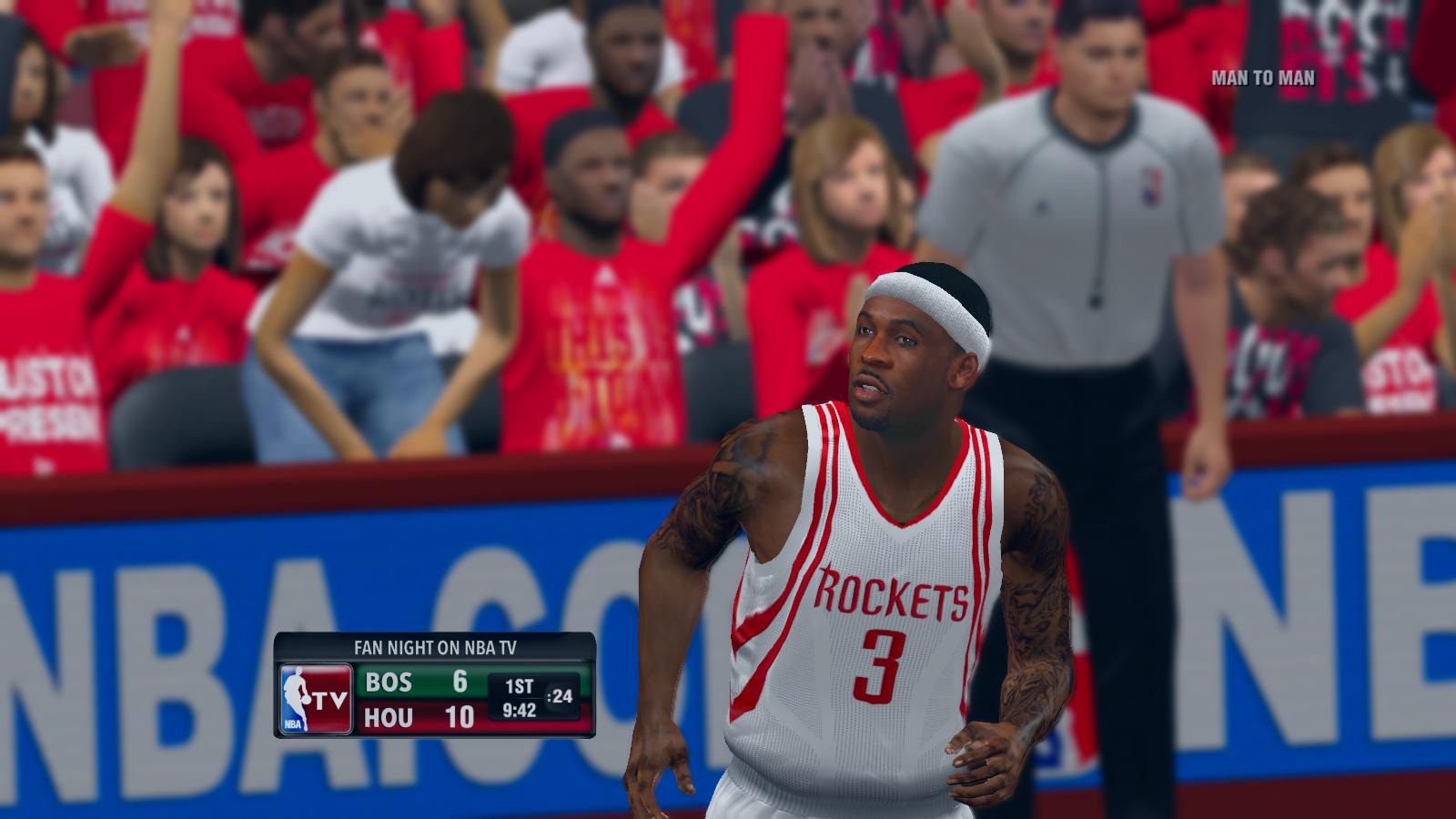The image depicts a dynamic moment from a basketball game, likely captured from a live broadcast on NBA TV during a "Fan Night" event. In the foreground, the prominent figure is a black player from the Houston Rockets. He is adorned in the team's signature white uniform with red accents, sporting a tank top and shorts, number three prominently displayed on his chest. His white headband stands out against his short, dark hair, and his well-groomed mustache and beard add to his distinct appearance. Tattoos are visible on both of his arms as he directs his gaze to the right, possibly towards the scoreboard.

The background reveals several rows of energized fans seated in red shirts, creating a vibrant sea of color in the bleachers. To the right of the center seating, a man who could be a referee stands out in his gray shirt and black pants, adding to the organized chaos of the scene. On the lower left corner of the image, a gray banner announces "Fan Night on NBA TV," accompanied by a small logo featuring a running figure with a basketball.

The scoreboard overlay in the bottom right corner provides real-time game information: "BOS 6 HOU 10" indicates the current score between the Boston Celtics and the Houston Rockets, with "First 9:42" showing the time remaining in the first quarter. The vibrant, action-packed scene is a snapshot of the energetic atmosphere typical of a live basketball game.